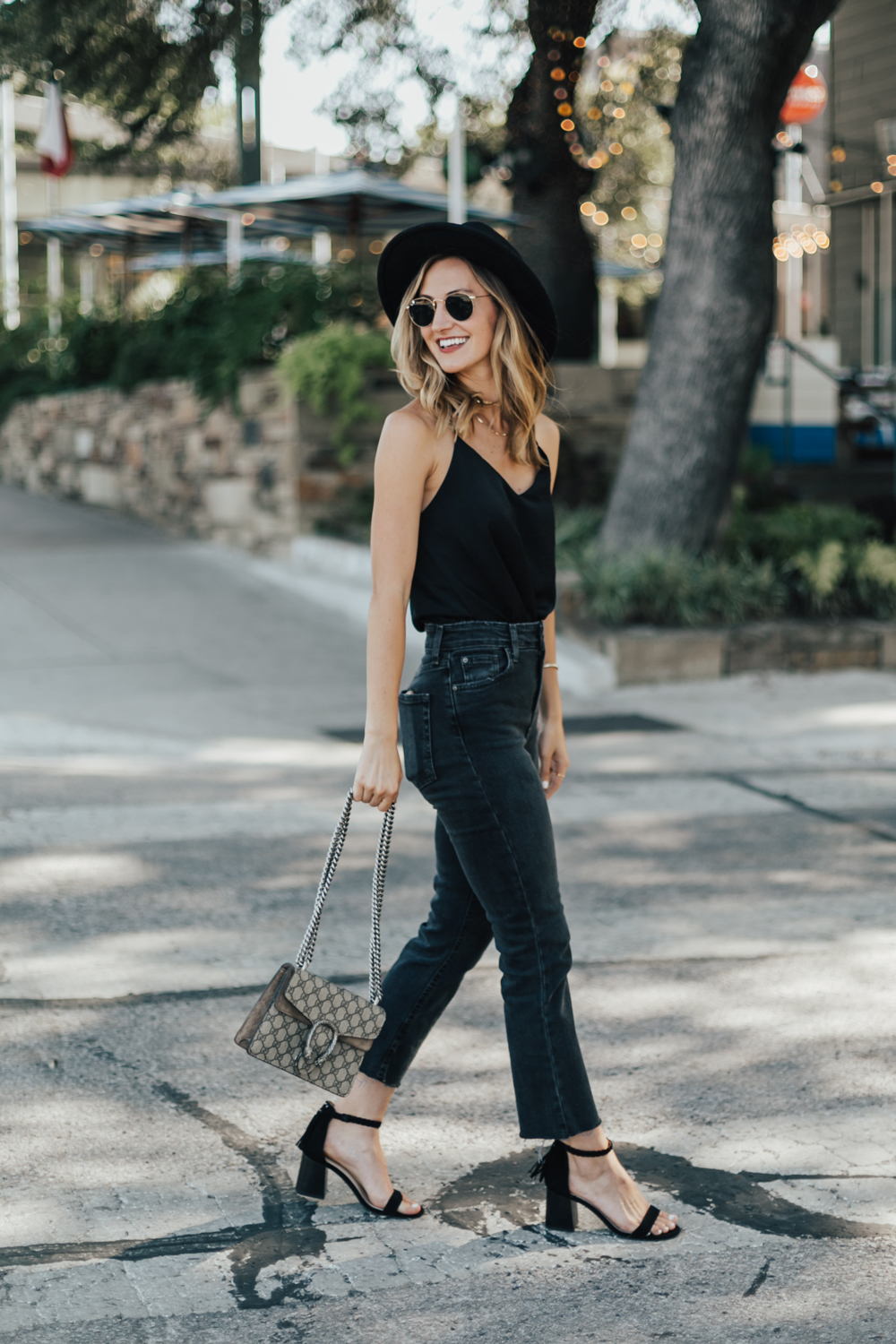This full-color, vertically aligned rectangular photograph features a young, slender, blonde-haired Caucasian woman walking along a concrete sidewalk on a sunny day. The professional model is dressed in a stylish black tank top with spaghetti straps, tucked into dark blue jeans, and complemented by high-heeled black sandals. She accessorizes with a broad-brimmed black hat, black round sunglasses, and carries a beige-patterned brown purse in her right hand, her left hand resting by her side with a visible bracelet. She is captured mid-stride, walking towards the right of the frame while glancing over her right shoulder to the left, smiling brightly.

The background includes various elements: two large tree trunks, one located in the upper right corner adorned with strings of lights, and lush green bushes surrounding a stone wall. A rail for a stairway is faintly visible, and higher up, there appears to be a white structure, potentially a covered shelter, reminiscent of a bus station. The backdrop blends natural elements and urban textures, highlighted by bright sunlight that bathes the entire scene.